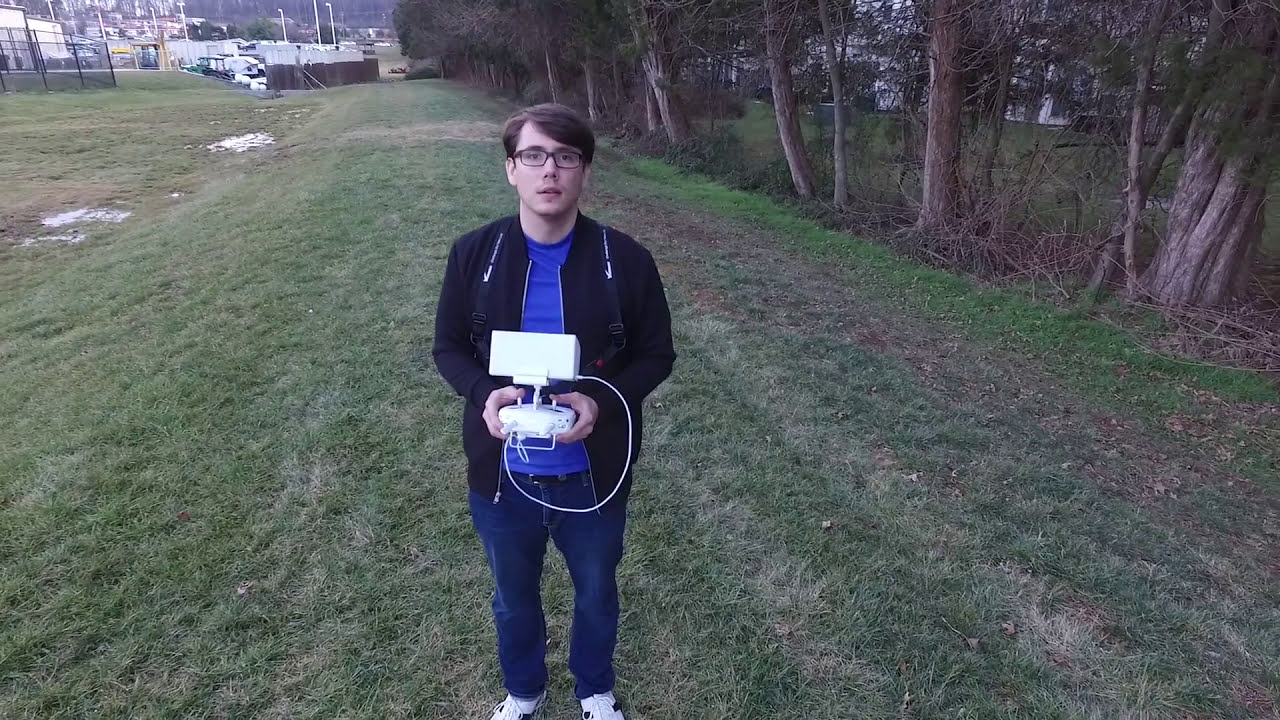The photograph captures a young white man standing in a green, somewhat patchy grass field, using a drone to take a picture of himself. He has parted, combed-over dark brown hair and is wearing black rectangular glasses. His attire includes a blue t-shirt underneath a black zip-up hoodie or jacket, dark blue jeans, and white sneakers with black stripes. He also has a black-and-white accented backpack on his shoulders. In his hands, he holds a white remote control, likely for the drone, equipped with a screen and wires. The scene is set outdoors, with a line of trees to his right, their rich green leaves contrasting with the brown trunks and branches, and some fallen leaves interspersed among the grass. In the background, partial views of buildings, a parking lot, and light fixtures can be seen, indicating a nearby complex. The grass appears recently cut, adding to the well-manicured look of the field.